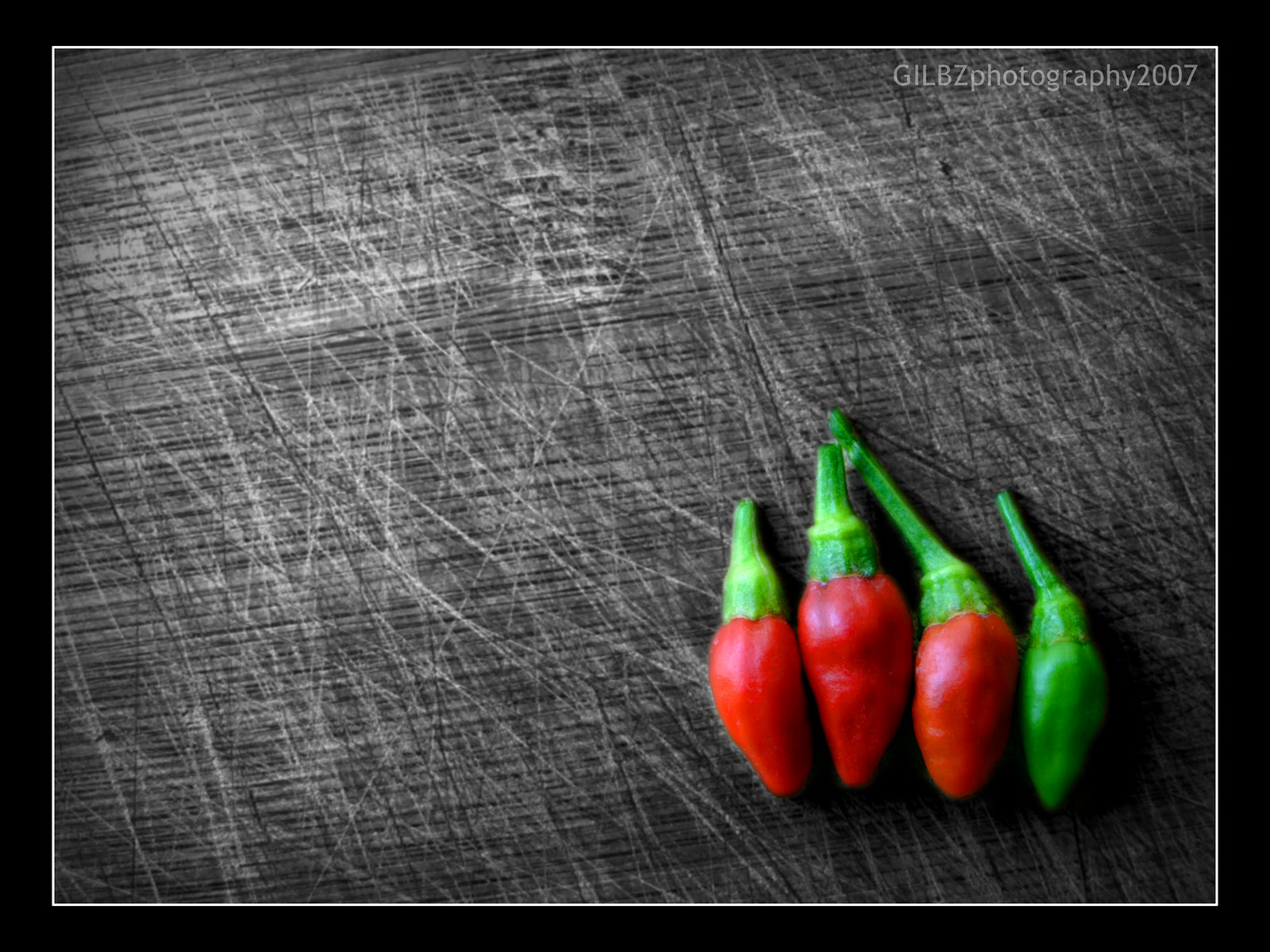The image features a stock photo style photograph with a thick black outline framing the scene. At its center, four highly saturated peppers are arranged linearly: three red peppers with green stems and one green pepper also with a green stem. These vibrant peppers, possibly chili peppers, have an unusually intense color saturation that contrasts sharply with the black and white, knife-scarred wooden surface beneath them. This background seems deliberately edited to be monochrome, emphasizing the vivid colors of the peppers. The overall effect is enhanced by a diffuse glow around the peppers, adding a slightly blurred, dreamy aura. In the upper right-hand corner, a watermark reads "GILBZ Photography 2007" in semi-transparent white lettering.